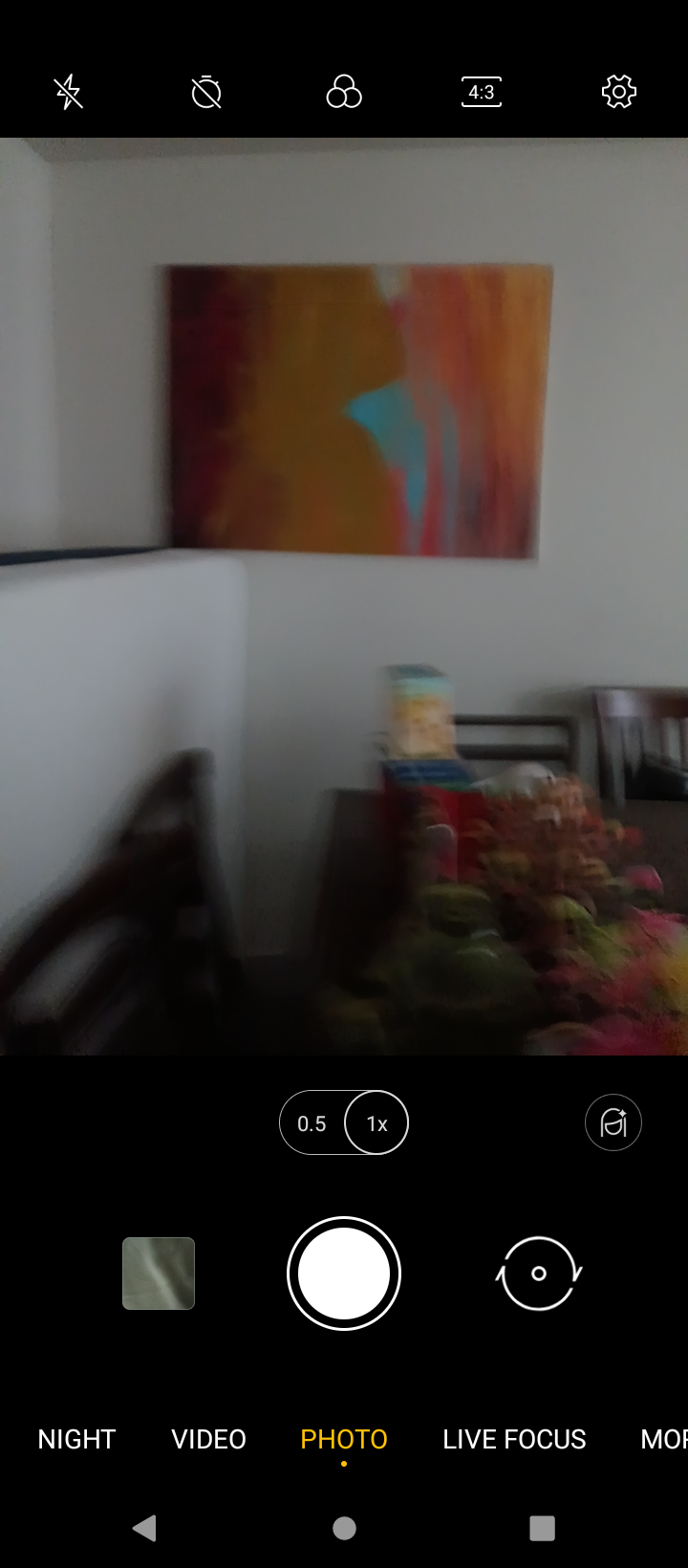The image depicts a phone screen in camera mode. At the bottom of the screen, there are various mode options: Night, Video, Photo, Live Focus, and Mode. The 'Photo' option is highlighted in orange, indicating it is the current selection, while the other options remain in white text. Just above these mode options, there is a central white circle, outlined in black with a thin white line around it, accompanied by additional icons.

The camera viewfinder shows a white wall adorned with an abstract art piece. This artwork predominantly features shades of orange and red, with a striking aqua blue section at its center. Below the artwork, there appear to be some indistinct chairs or objects, mostly in shadow, making it difficult to discern their exact nature. The overall scene captured by the camera is a blend of bright and vibrant art against a dimly lit foreground.